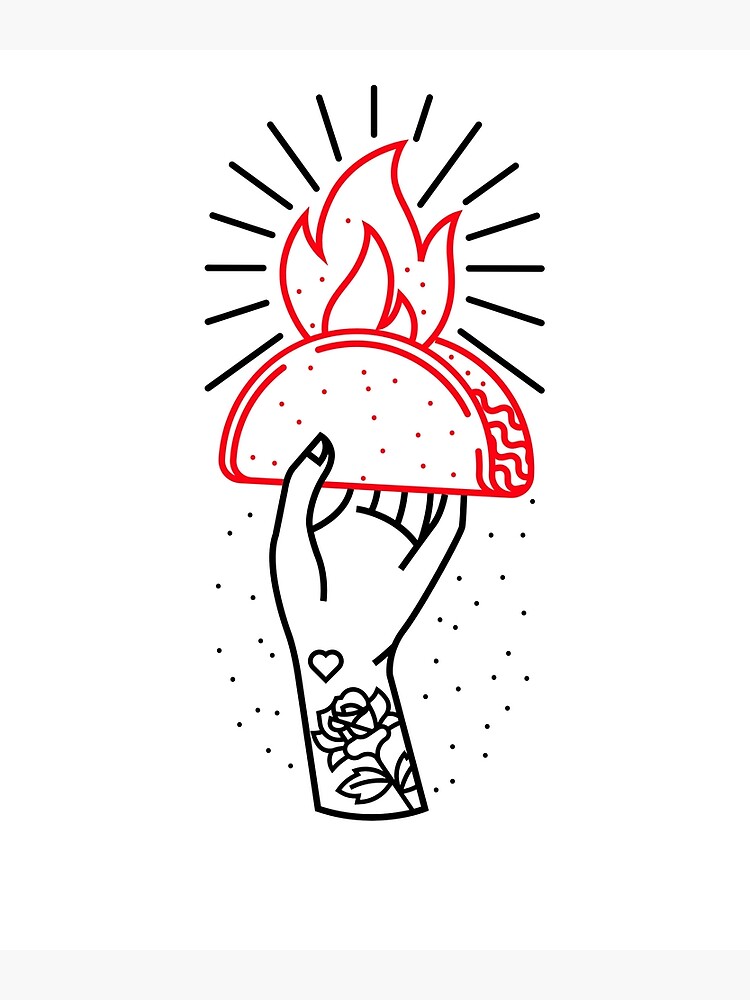This image is a detailed line drawing featuring a woman's hand and wrist. The hand is animated, showing the thumb in the front and four fingers at the back, extending just a few inches below the wrist. On the wrist, there is a black and white tattoo of a rose, placed below a small heart. The wrist and lower hand are decorated with numerous black dots. The hand grasps a red, stylized object resembling the top part of the Statue of Liberty’s torch or a taco—with red flames emanating from it, suggesting intense heat or spiciness. Surrounding the flames are black radiating lines, totaling fifteen, which emphasize the dynamic nature of the drawing. The entire illustration is set against a white background.